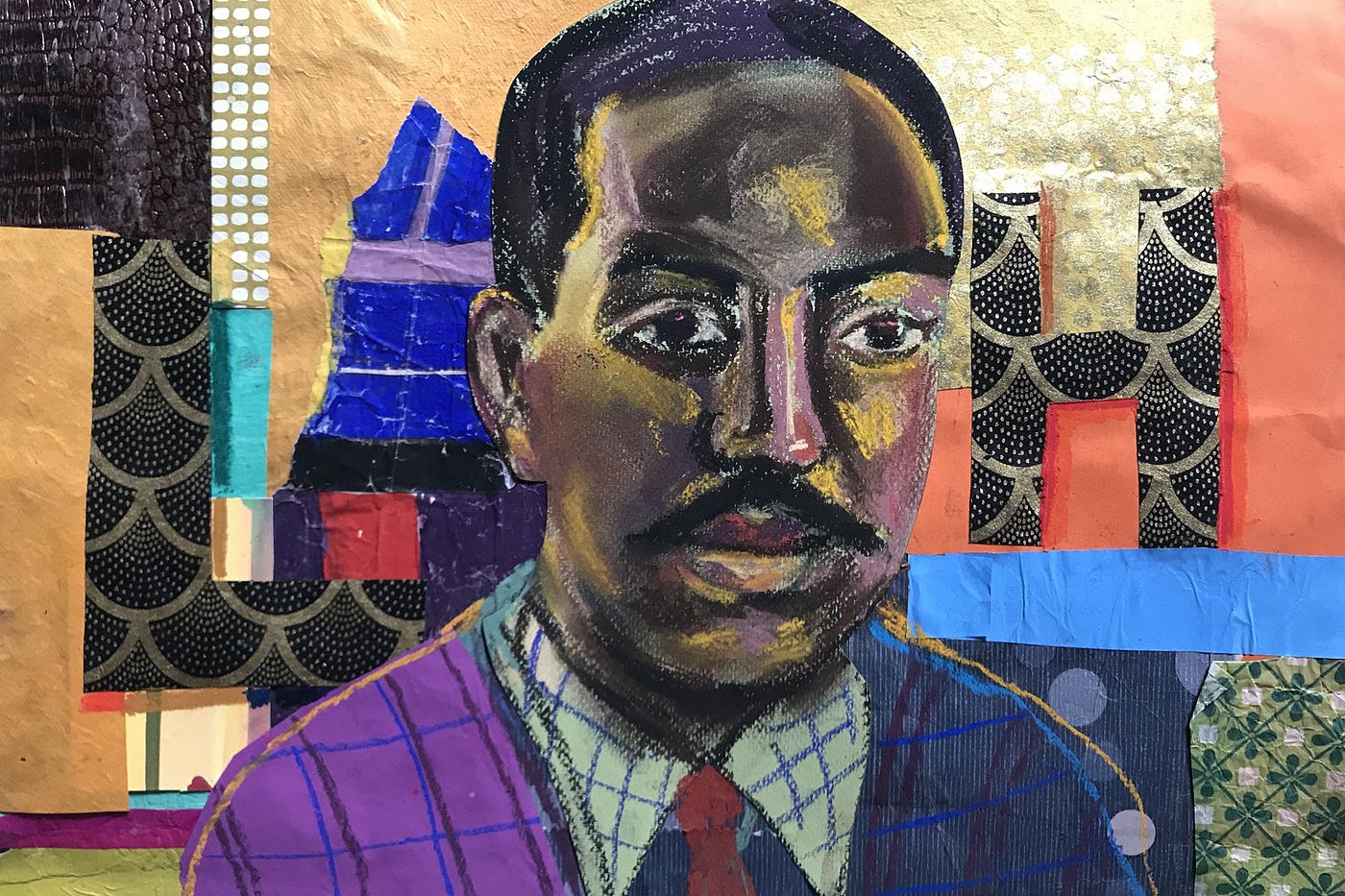The image is a detailed, mixed-media portrait of an African-American man. He appears to be around 50 years old, with very short hair and a mustache, holding a neutral expression as he looks straight ahead. His attire is a patchwork of vibrant patterns—he wears a unique shirt that seems assembled from pieces of different flannel designs: the left shoulder is purple, the right side is black and blue, and the center is white and blue. Complementing his eclectic shirt, he wears a striking red tie. The background is an intricate collage featuring an array of colors and shapes: predominant tones include a large vertical brown section to the left, a salmon-colored area on the right with a blue stripe, and various other hues like light beige, clover green, purple, and black. The collage includes diverse elements such as floral designs, cut-out shapes resembling letters, and different wallpaper pieces like polka dots and solid blocks, contributing to an abstract, modern art feel. The overall medium of the artwork appears to be a combination of oil paint, crayon, and pastels, giving it a textured, layered look.